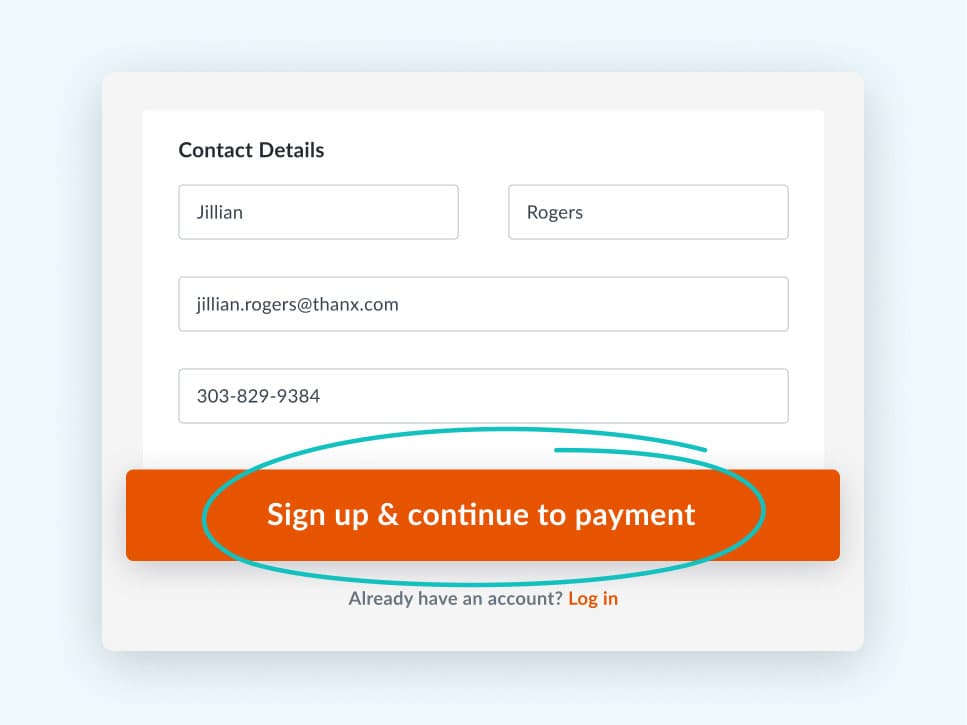The image appears to be a screenshot taken to highlight specific details. It features a light blue background with a white pop-up box in the center, outlined in a subtle gray border. In the upper left corner of the white box, the heading "Contact Details" is prominently displayed. Below this heading are two adjacent rectangular fields: the first contains the first name "Jillian" and the second contains the last name "Rogers." 

Further down, a longer rectangular field displays the email address "Jillian.Rogers@thanks.com" (with "thanks" spelled as "thanx"). Beneath the email field, another rectangular box contains the phone number "303-829-9384."

At the bottom of the white box is an orange button that spans the entire width of the pop-up. The button features white text that reads "Sign up and continue to payment." This entire section, including the button, is highlighted by a teal-colored circle, presumably drawn with a marker to indicate its importance.